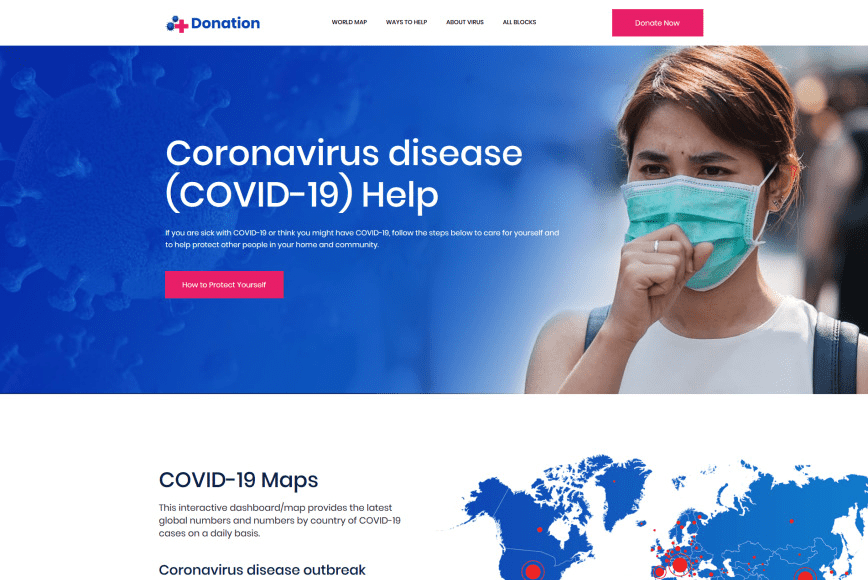The image appears to be a screenshot from the Red Cross website, which is themed around COVID-19 awareness and support. At the top of the page, the word "Donation" is prominently displayed alongside the iconic Red Cross emblem, emphasizing the importance of contributions in these times. Below this header, a vibrant red "Donate Now" button is positioned for easy access.

Dominating the upper section of the page, a blue background features a woman with brown hair and light skin, wearing a green mask, symbolizing protective measures against the virus. Text next to her reads, "Coronavirus Disease (COVID-19): Help," urging visitors to seek guidance. The text further advises, "If you are sick with COVID-19 or think you might have COVID-19, follow these steps below to care for yourself and help protect other people in your home and community." Adjacent to these instructions is another red button labeled "How to Protect Yourself" in white text, offering practical advice.

Beneath this informative section lies an interactive map titled "COVID-19 Maps". This dashboard provides up-to-date global statistics and country-specific numbers on COVID-19 cases. The world map is color-coded, with blue representing the land and white indicating water, while red spots highlight areas of significant outbreaks, helping users track the spread of the virus effectively.